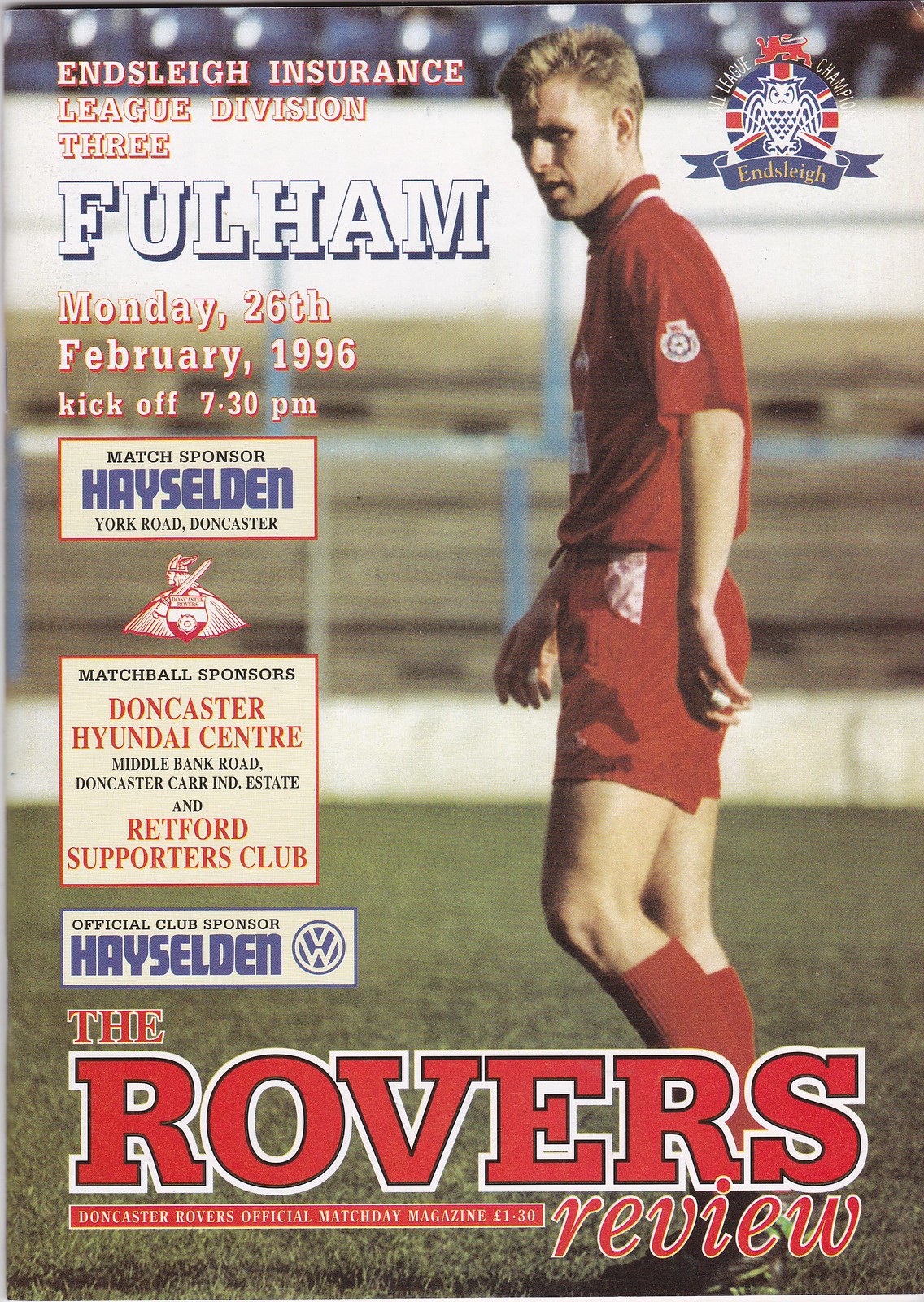This is a 1996 game day magazine that you might purchase at a soccer match. The cover features a large photo of a soccer player in a red uniform, staring down the field. Surrounding the image are various details and sponsorship logos. The top left text reads: "Ensley Insurance League Division III, Fulham, Monday, February 26, 1996, kickoff 7.30pm." Additionally, there are sponsorship acknowledgments such as "Match Sponsor: Hazleton, York Road, Doncaster" and "Match Ball Sponsors: Doncaster Hyundai Center, Middlebank Road, Doncaster Car, Industry Estate, and Redford Supporters Club." The middle prominently displays the team logo, which resembles a shield and a cape. The bottom portion of the page features a bold title in large red text with a white border, stating, "The Rovers Review: Doncaster Rovers Official Match Day Magazine," priced at $1.30.